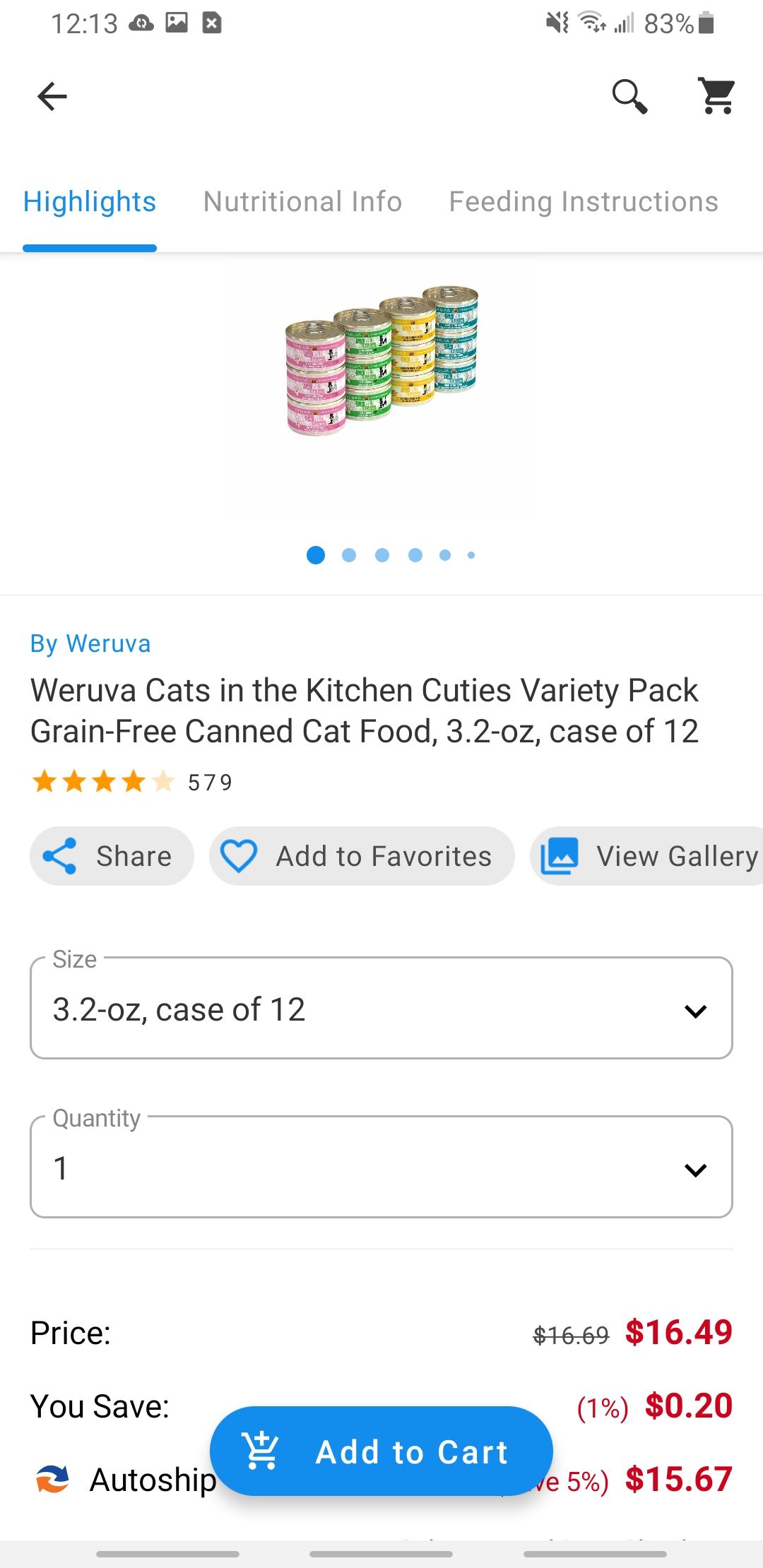Here is the cleaned-up and detailed caption for the given image:

---

This portrait-mode screenshot presents a comprehensive product overview for a cat food item. 

- **Status Bar:** The top left corner displays the time as 12:13, while the top right corner shows the battery charged at 83%.

- **Navigation Bar:** Just below, the left side features a black back arrow, and the right side includes search and cart icons.

- **Tabs:** The following row contains three headings: "Highlights," "Nutritional Info," and "Feeding Instructions." "Highlights" is highlighted in blue and underlined, indicating the current active tab.

- **Product Image:** The main portion of the screen showcases an image of stacked cat food cans organized in four stacks and three rows, displaying cans in pink, green, yellow, and blue colors. Below the image, there are six dots that progressively decrease in size from the first to the last. The first dot is the largest and is colored blue, suggesting more images can be viewed by scrolling.

- **Product Information:** Below the image is the product branding by "Weruva," typed "W-e-r-u-v-a" and presented as a clickable blue link. The product name is "Weruva Cats in the Kitchen Cuties Variety Pack, Grain-Free, Canned Cat Food, 3.2 oz, Case of 12."

- **Review & Rating:** The product has been rated four stars out of five, based on 579 reviews.

- **Action Buttons:** There are three buttons with dark gray backgrounds beneath the review section: a share button, an add-to-favorites button, and a view-gallery button.

- **Purchase Options:** A dropdown menu form follows, displaying the size option as "3.2 oz Case of 12" and the quantity set to one. The price is listed at $16.49, with an original price of $16.69, reflecting a 1% (20 cents) savings. 

- **Add to Cart:** At the bottom, there is a prominent blue "Add to Cart" button.

---

This caption provides a detailed and structured description of the screenshot, making it clear and informative.